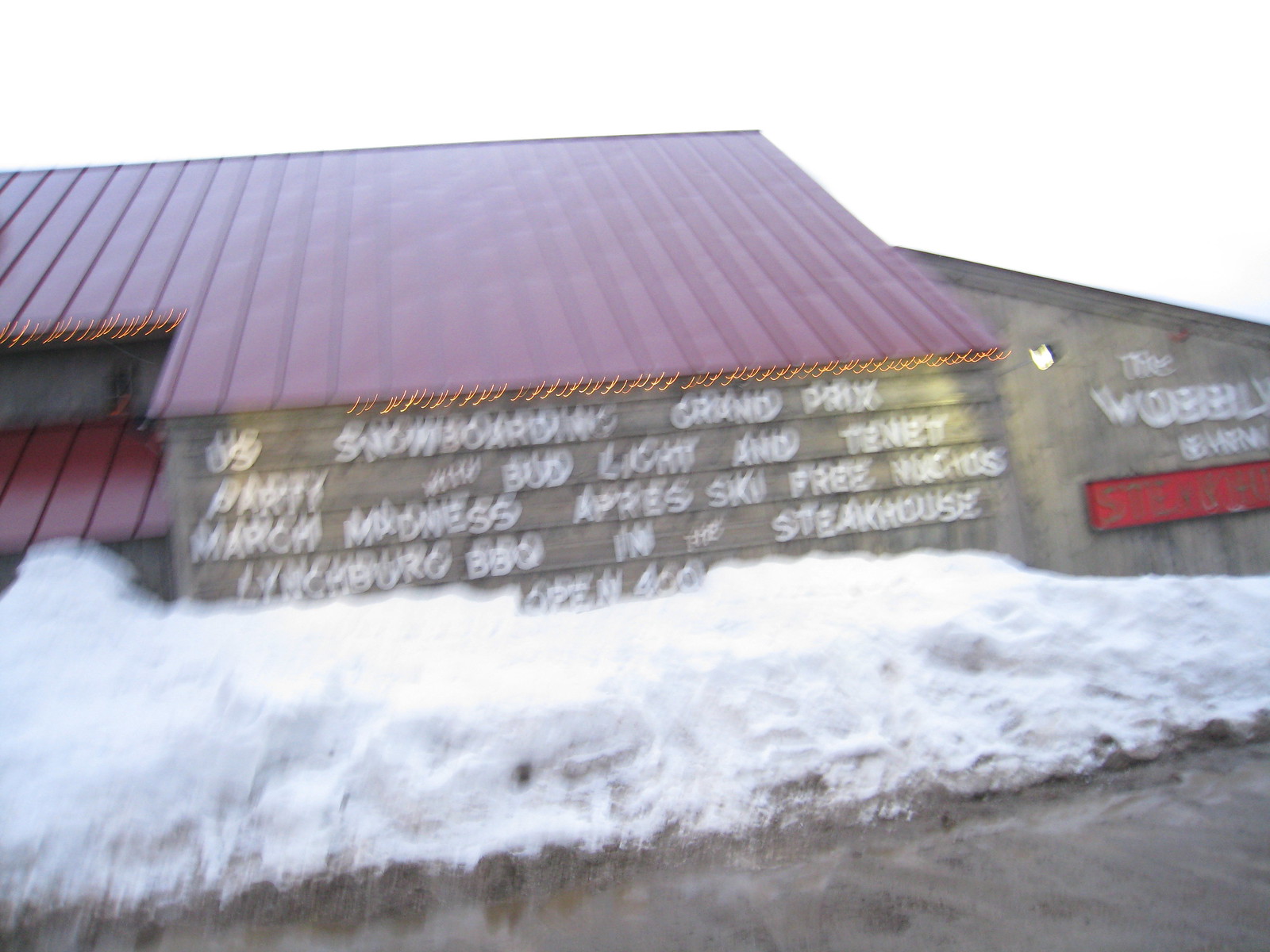This photograph captures the exterior of a rustic building set against a grayish, muddy ground that transitions into a buildup of white snow in front of the structure. The building, characterized by its gray wooden facade, features a prominent, angled red roof. On the right side of the building, signage reads "The Wobbly Barn." Despite the blurry image, legible white print on the signage announces various events, including the 'U.S. Snowboarding Grand Prix Party with Bud Light' and 'Tenant March Madness.' Additional text promotes an 'Après-ski' event offering free nachos at a Lynchburg BBQ located in the steakhouse, which opens at 4 PM.